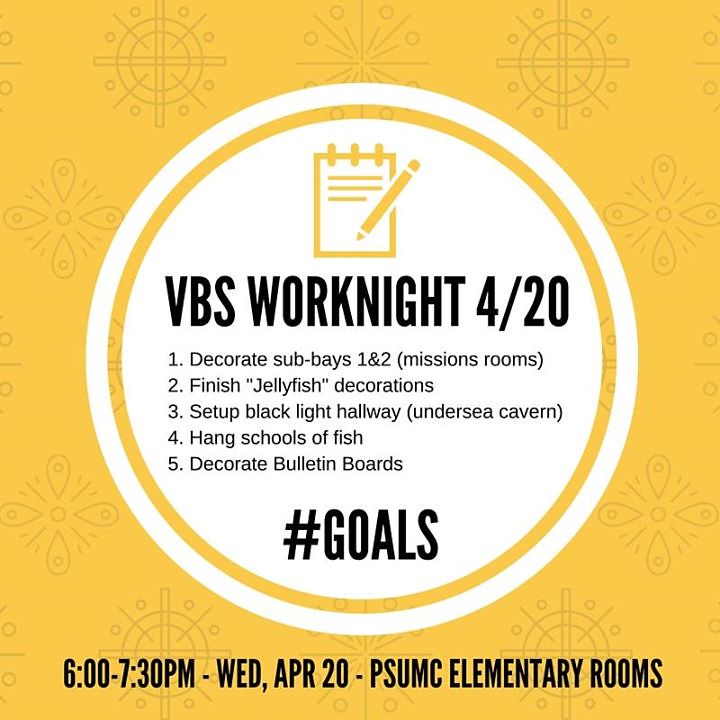The digital image features a vibrant, mustard-yellow background adorned with faint, symmetrical geometric patterns, including circles, crosses, and star-like shapes. Dominating the center is a large white circle with a cartoon-style outline of a yellow notebook and pencil positioned at its top. Below this, the heading "VBS Work Night 4/20" is prominently displayed in large black font. Underneath the heading is a list of five tasks: 1) Decorate Sub Bays 1 and 2, Mission Rooms, 2) Finish Jellyfish Decorations, 3) Set Up Blacklight Hallway Undersea Cavern, 4) Hang Schools of Fish, and 5) Decorate Bulletin Boards. In much larger black font, the phrase "#GOALS" is emphasized. Centered at the bottom of the white circle, the event details are clearly stated: "6:00 to 7:30 PM - Wednesday, April 20th, PSUMC Elementary Rooms."